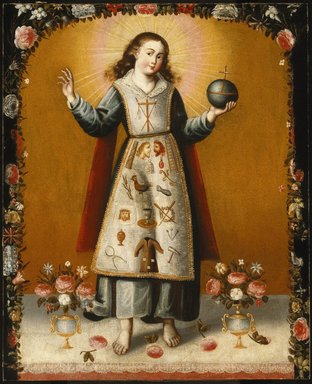This medieval-style painting portrays a saintly woman standing at its center, possibly representing Joan of Arc. She is draped in a flowing red cape over a gray gown and light blue pants, and a gold-trimmed, white apron adorned with intricate religious iconography sets her apart. On her apron, detailed depictions of chisels, tongs, birds, men, wheat, chalices, and an image of Jesus with a crown of thorns emphasize her sanctity and purpose. The apron also displays Christ’s head dripping blood and other holy symbols. A gold cross adorns her chest, emphasizing her holy stature.

In her left hand, she reverently holds a silver orb topped with a cross, reminiscent of the holy hand grenade from Monty Python's tale, symbolizing divine power and authority. Surrounding her feet are several flower vases, each holding three roses, contributing to the solemn and serene atmosphere.

Her presence is framed by a black border embellished with floral designs, roses, crosses, and doves, rendered in red, gold, and silver. The background behind her features a golden-brown wall that creates a halo effect, illuminating her head and enhancing her saintly aura. The entire composition is rich in gold, white, gray, and black tones, emphasizing both the divine and historical significance of the subject.